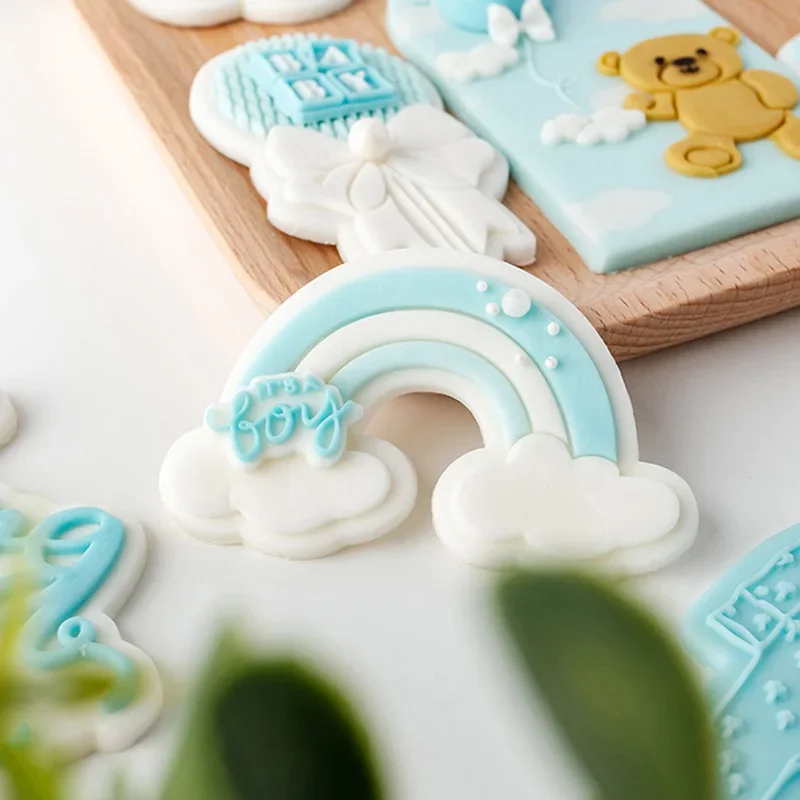This is a detailed and vibrant image capturing an array of beautifully decorated cookies, likely prepared for a baby boy's shower. At the center is a whimsical cookie featuring a cheerful rainbow in alternating light blue and white stripes, capped with fluffy white clouds. Inscribed on one cloud in light blue letters is the phrase "It's a boy." Adorning the top right corner of this rainbow cookie are delicate pearls. Surrounding this standout piece is a charming assortment of other cookies displayed on a wooden cutting board placed on a white surface. Among them, there's a delightful teddy bear clutching a balloon, soaring amidst blue skies and white clouds. Another cookie, resembling a rattle, spells out "baby" in playful block letters against a blue and white backdrop. Additionally, the corners of the image reveal glimpses of other cookie edges, hinting at more blue-themed designs, with one peeking out to say "boy." The lower portion of the photo, though blurry, completes the scene with the subtle presence of green plants or leaves, enhancing the festive yet serene ambiance of the celebration.